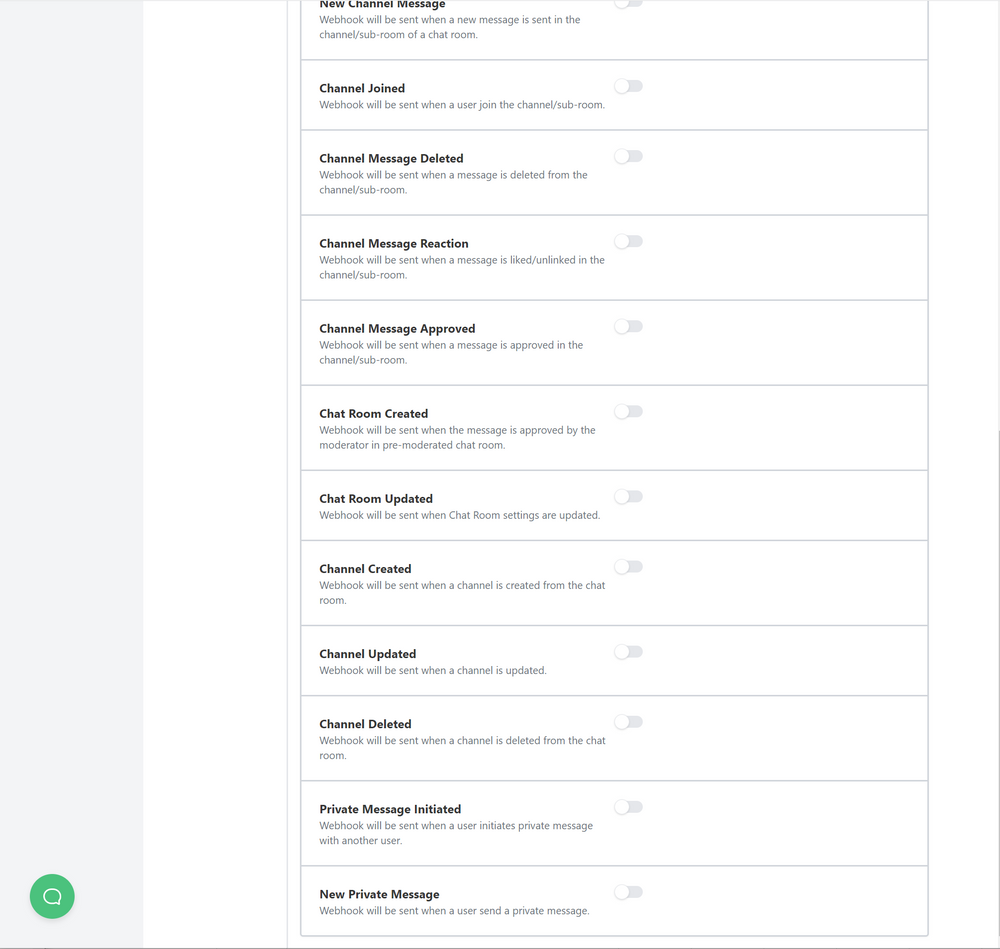The image depicts a predominantly white settings webpage, likely from a chat room service or a related platform. The page is clean and minimalist, with a series of horizontal setting boxes that stand out against the white background. Each box comprises a bolded, black title on the left followed by a descriptive text in lighter, grayish font underneath. Central to each setting box is a slider mechanism that can be toggled to the right to enable the corresponding setting.

From top to bottom, the first setting is titled "New Channel Message" in bold, black text. Below this, the description reads: "A webhook will be sent when a new message is sent in the channel/subroom of a chat room."

The next setting is "Channel Joined," also in bold, black text with its description stating: "A webhook will be sent when a user joins the channel/subroom."

Following that is "Channel Message Deleted" in bold, black text, and its accompanying description explains: "A webhook will be sent when a message is deleted from the channel/subroom."

Based on the settings listed, it can be inferred that the term "webhook" represents an action triggered by various events within the chat room or subroom, rather than the name of the website itself.